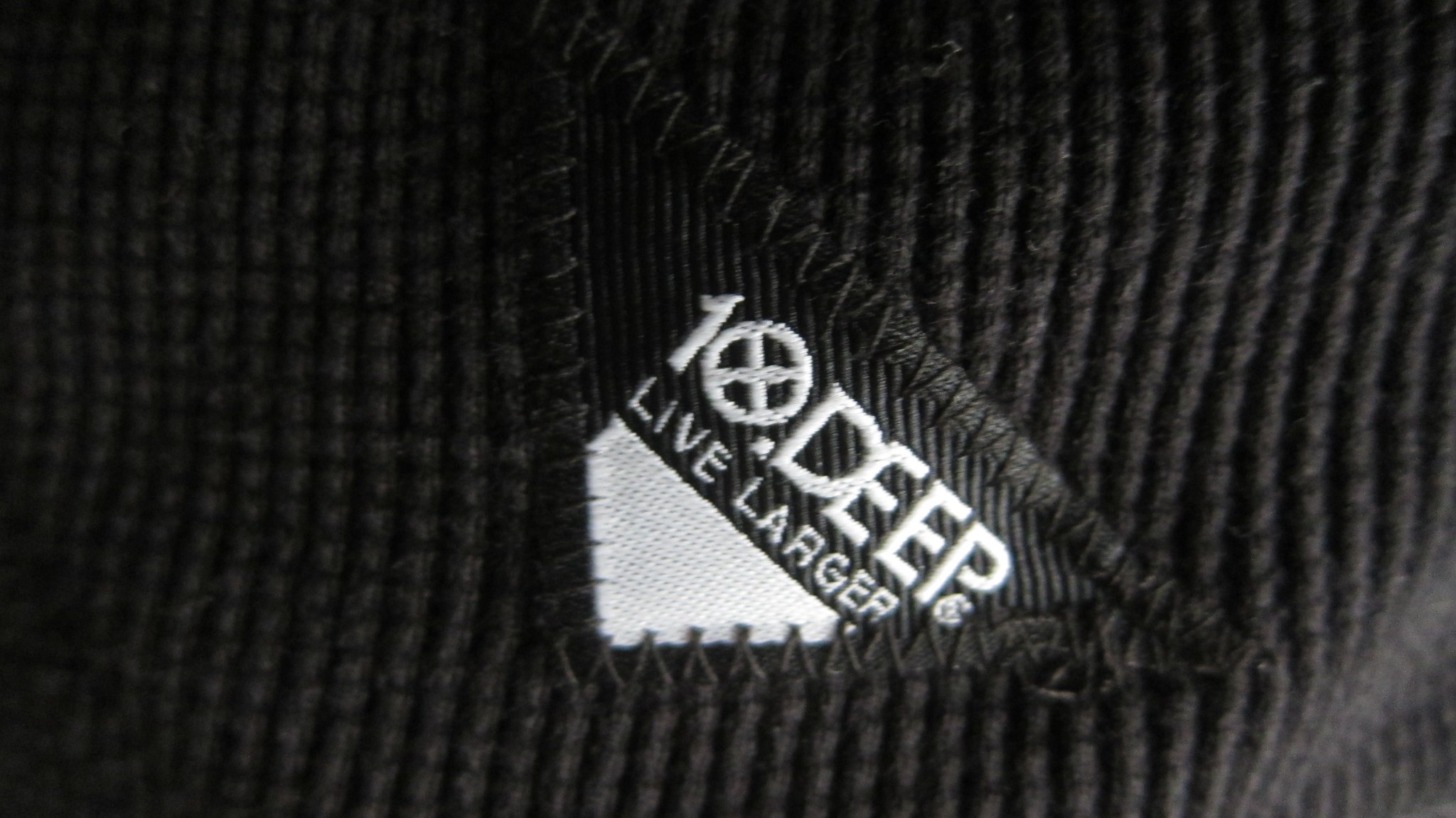The image is a close-up photograph showcasing a black fabric material that appears to be medium weight, possibly from a sweater. The fabric is intricately textured with vertical and horizontal stitching, hinting at being machine-sewn. The focal point of the image is a sewn-in, right-angled triangle label, centrally positioned on the fabric. The triangle features a dark black and gray striped pattern and is bordered with black thread. The bottom section of the triangle is white. On this label, there's bold white text that reads "10.DEEP". The '0' in '10' has two lines intersecting it, forming an 'X'. Below this, in slightly smaller capital letters, it states "LIVE LARGER". The bottom-right corner of the image fades to a lighter white, suggesting light exposure.